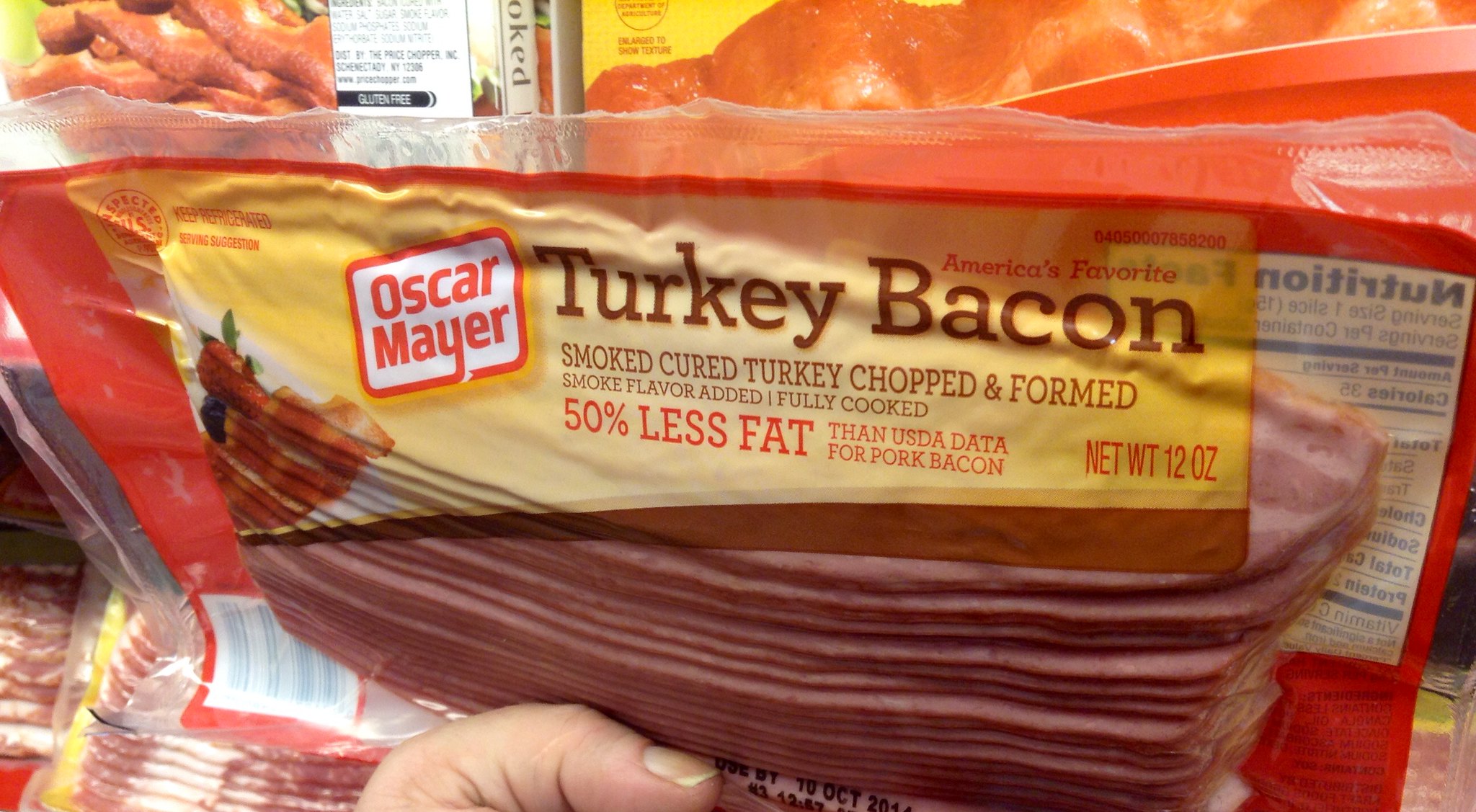In the image, a person is holding a package of Oscar Mayer turkey bacon, wrapped in clear plastic shrink wrap. The package prominently displays several labels, including "turkey bacon," "smoked," "cured," "chopped and formed," "smoke flavor added," "fully cooked," and "50% less fat than USDA data for pork bacon." The label also notes a net weight of 12 ounces and proudly claims to be "America's favorite." Through the transparent bottom of the packaging, you can see the pink, meat-like slices of the turkey bacon. In the background, there are several boxes of other types of bacon. To the left of the package, a plate holds what appears to be real pork bacon, providing a visual comparison. Also visible in the image is the person's thumb gripping the package.